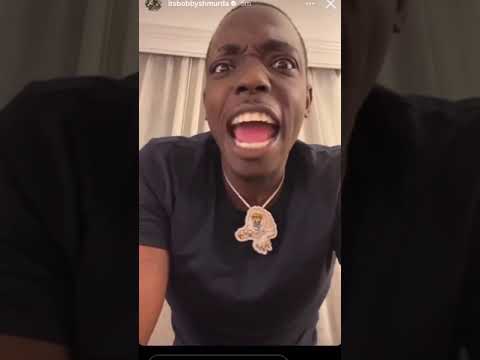This image is a compressed and pixelated screenshot from an Instagram reel or live stream featuring Bobby Shmurda, a young African American man with dark brown skin and a fade haircut. He is wearing a black short-sleeved shirt and a necklace with a pendant that seems to resemble a character or a large beast, though the exact details are unclear. Bobby is smiling broadly, showcasing his white teeth adorned with gold grills. His right eye is slightly open while his left eye appears more closed. The background includes a white curtain and ceiling, possibly indicating an indoor or hotel setting. The image is framed with blown-up duplicates of Bobby on the left and right sides. Visible at the top is the username "It's Bobby Shmurda" along with a profile picture and a white verification checkmark. Additionally, his right hand seems to be partially off-screen, potentially flashing a peace sign.